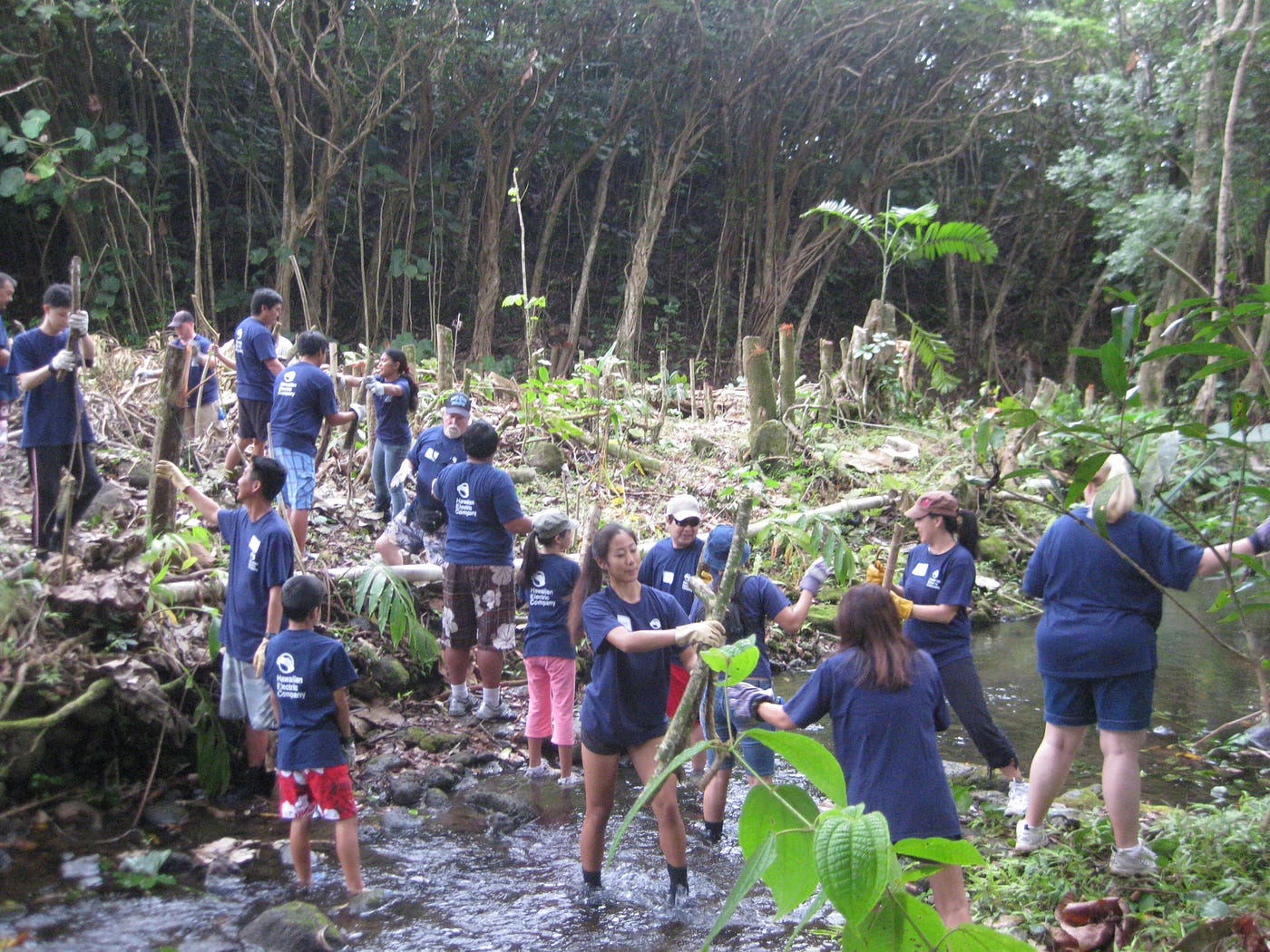In this outdoor photograph, around 16 to 20 people—comprising both young volunteers and a few adults—are actively engaged in a clean-up effort within a lush forest. The background showcases tall, dense trees with thin brown trunks and vibrant green leaves. Centered in the image is a flowing creek or small pond, where some volunteers stand in the water, while others work on adjacent land. The group is uniformly dressed in dark blue t-shirts, complemented by various types of shorts, jeans, or pants. Distinctive clothing items include pink capri pants, jean shorts, and red or gray swim trunks. Many participants are equipped with work gloves in shades of white or gray and some wear hats. They are seen picking up large sticks and branches, possibly remnants of recently cut-down trees, and engaging in conversation as they carry out their tasks.